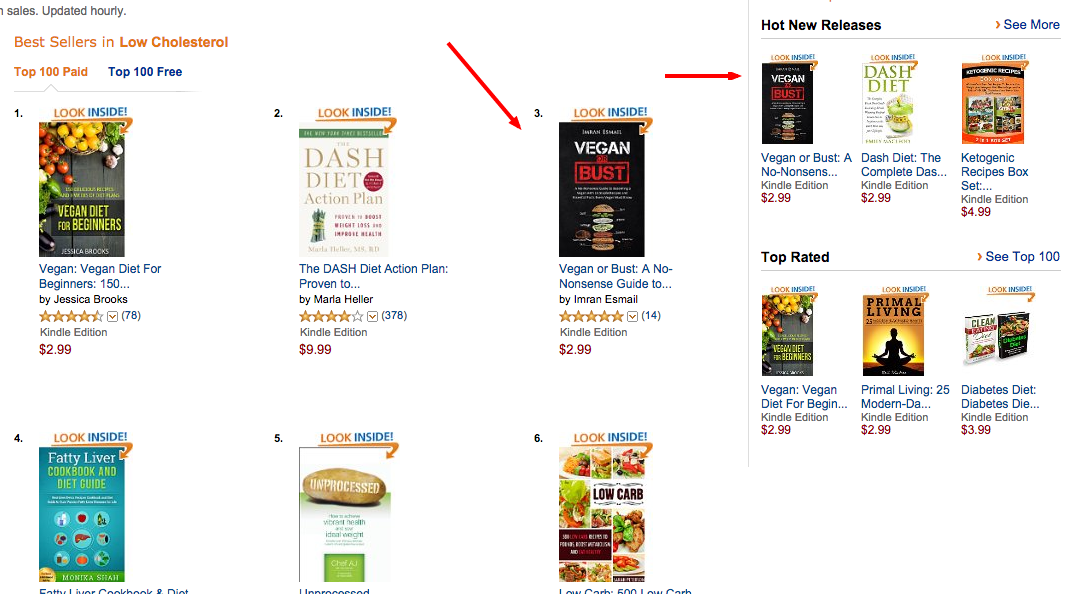This screenshot from Amazon displays the "Best Sellers in Low Cholesterol" section of their books’ search results page, set against a white background. At the upper left corner, written in a distinctive gold font, it says "Best Sellers in Low Cholesterol," followed by "Top 100 Paid" in gold and "Top 100 Free" in blue.

Taking up around two-thirds of the left side of the page are six book titles, arranged into two rows with three books per row. From left to right in the top row, the titles are: "Vegan Diet for Beginners," "DASH Diet Action Plan" with a white cover, and "Vegan or Bust: A Nonsense Guide to…" (the rest of the title is obscured). In the bottom row, the titles are: "Fatty Liver Cookbook and Diet Guide" with a blue cover, "Unprocessed" featuring a large Idaho potato with the title written in white font on the potato, and "Low-Carb" with images of various foods such as salads and sandwiches.

On the right side of the page, a smaller section highlights "Hot New Releases." Some duplicated titles here include "DASH Diet Action Plan" and "Vegan or Bust." Additional titles featured are "Ketogenic Recipe Box Set" with an orange background, "Vegan Diet for Beginners," and "Primal Living," which is depicted with a silhouette of a person sitting cross-legged in a yoga pose.